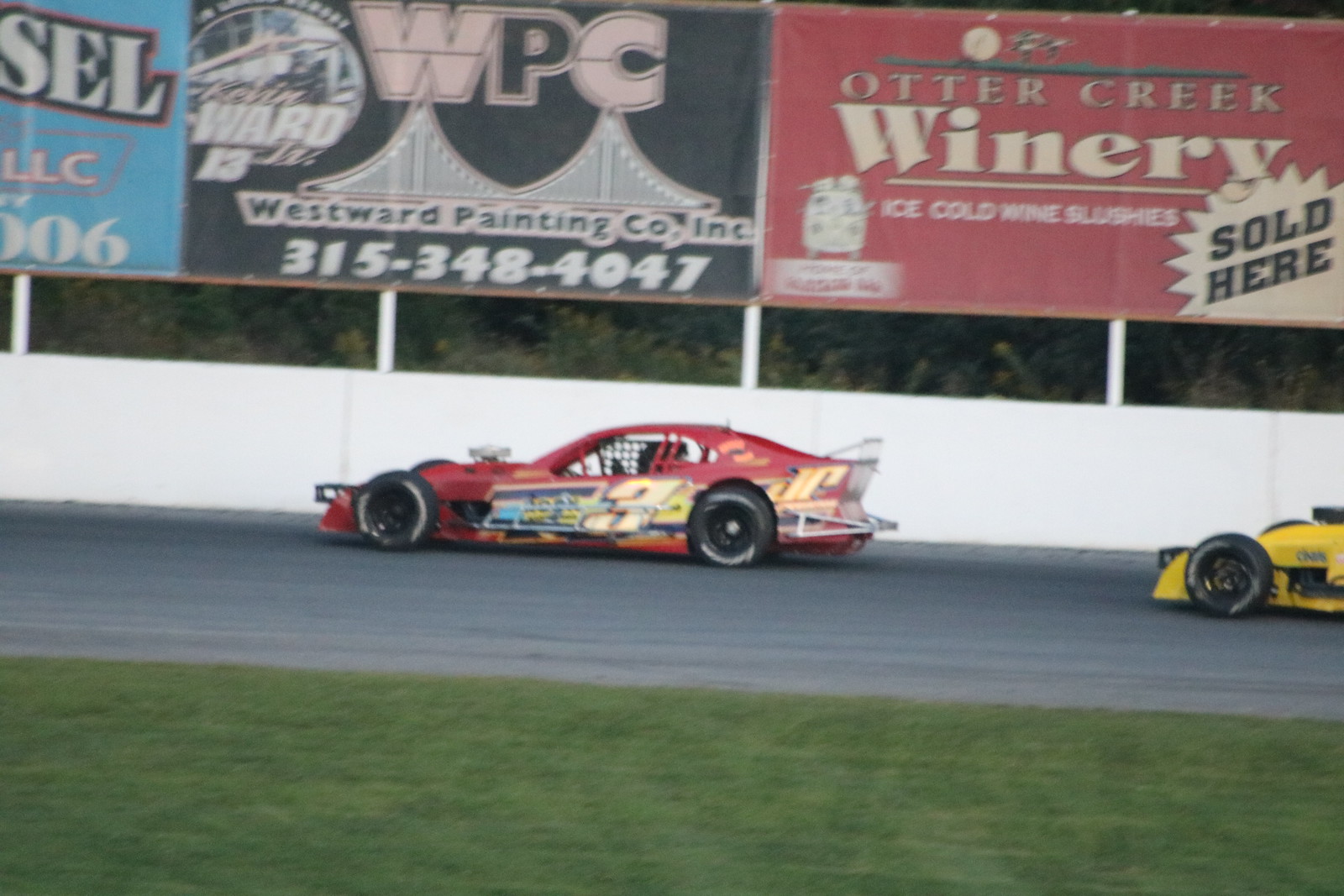This horizontally aligned rectangular photograph captures the action of a race car speeding down a racetrack. In the foreground, vibrant green grass frames the image, leading the eye to the main scene. The focus is on a red race car prominently displaying the number 34 in bold yellow on its door. Additional markings include "JP" in yellow on the rear fender and another insignia in gold and blue. The car's engine is exposed, protruding from the hood to optimize air intake, and netting can be seen on the driver's side window. Adjacent to this vehicle, the front end of a yellow race car is visible on the right side of the image, trailing closely behind. The red car races beside a white wall, topped with various advertising signs. Notable adverts include a sign for WPC, Westward Painting Co., Inc., with its phone number, and a red sign promoting Otter Creek Winery, highlighting their Ice Cold Wine Slushes. In the upper left corner, a partial view of a blue sign reads "S-E-L," although the remainder is obscured. Beyond the wall, a backdrop of trees adds a sense of depth, while the overall image maintains a slightly blurry, dynamic effect, enhancing the sense of speed and movement.